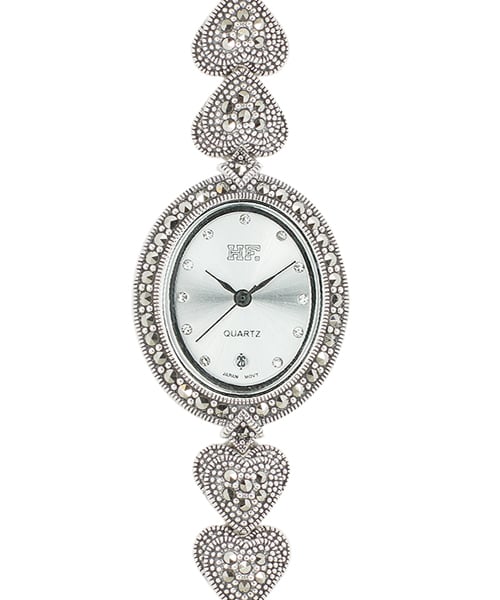The image depicts a luxurious silver and black timepiece, ideal for a retail or auction setting, set against an all-white background. At the center is an oval watch face with black hour, minute, and second hands, all encircled by gem-studded markings in place of numbers. The watch face features the initials "HF" below the 12 o'clock position and the word "quartz" above a small date window displaying the number "26." The band is composed of intricately connected hearts, each encrusted with rhinestones, creating an elegant design. The top of the image highlights two upside-down hearts, while the bottom features two right-side-up hearts, completing the opulent band.